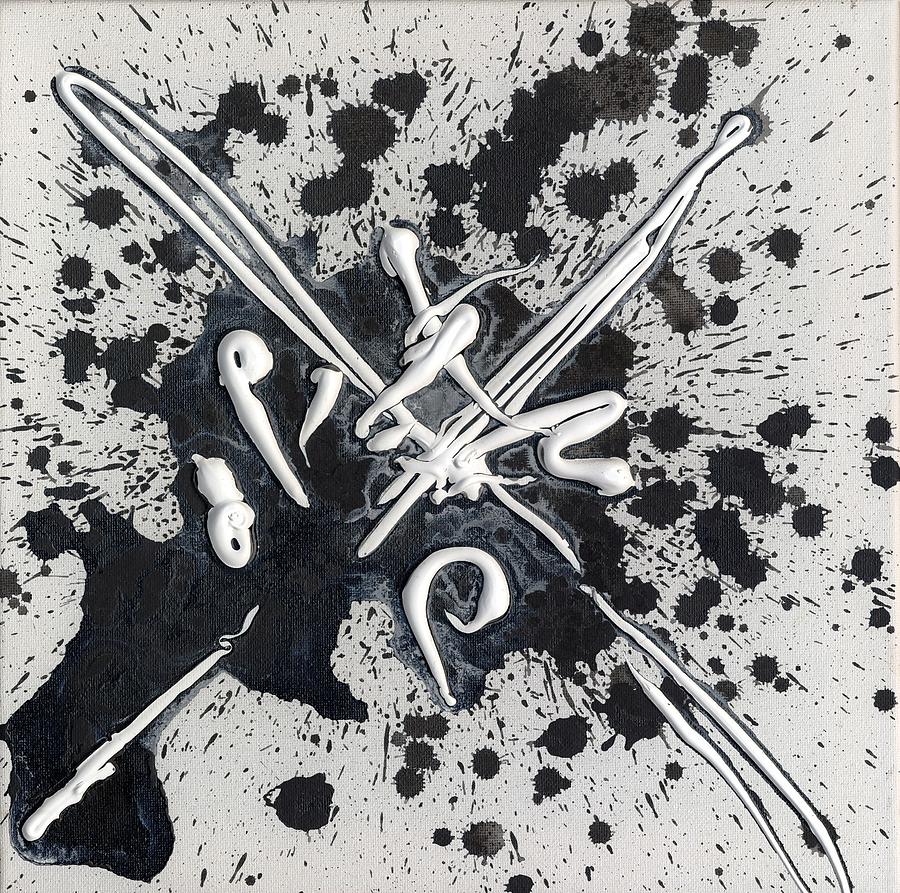This image features a square black and white abstract painting on a light gray, textured canvas. Dominating the composition are chaotic black ink splotches and paint drippings, which appear to have been haphazardly splashed across the canvas. Central to the image is a stark, conspicuous 'X' formed by thick swipes of black paint, giving the impression of paint being energetically flung back and forth. Surrounding this central black zone are large splotches and smaller splashes, creating a sense of dynamic motion. Intertwined amongst the black elements are fine, white paint swirls, some thick and others thin, meandering in various directions. These white strands loop and twirl intricately, infusing the central area with a swirling, almost chaotic beauty, like an artful cake decoration. The texture of the underlying canvas is discernible throughout, adding a tactile dimension to this visually striking piece.